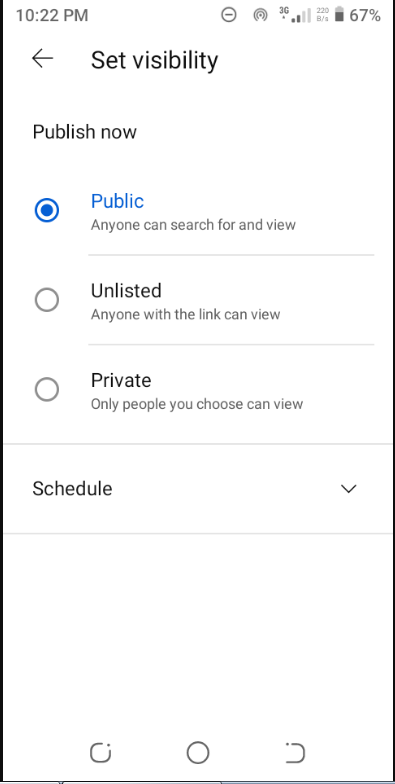This image is a detailed screenshot from a mobile device, captured in portrait orientation with black borders along the top, bottom, left, and right sides. The top of the screenshot does not have a border, and the image is against a white background, appearing significantly taller than it is wide, maintaining the typical proportions of a smartphone screen.

At the top of the screen, there is a grey font displaying the time "10:22 PM," followed by a sequence of icons: a "Do Not Disturb" symbol, a "Mobile Hotspot" icon, a "3G" icon, and a network connection indicator showing 2 out of 4 bars. Additionally, there is text featuring "220" over the letters "B-A," accompanied by a vertical battery icon indicating a 67% charge with a dark grey meter.

Below the status bar, a black left-pointing arrow is situated next to a header that reads "Set Visibility." Directly beneath this header, the text "Publish Now" is displayed, followed by three options with radio buttons: 

1. "Public, anyone can see, search for and view," which is selected and highlighted in blue with a filled blue circle.
2. "Unlisted, anyone can see with a link and view."
3. "Private, only people you choose can view."

Further down, the section is bordered in light grey and contains a "work schedule" dropdown option marked by a downward-facing caret. 

The bottom of the screenshot is filled with some white space, followed by familiar icons representative of standard phone interface functions.